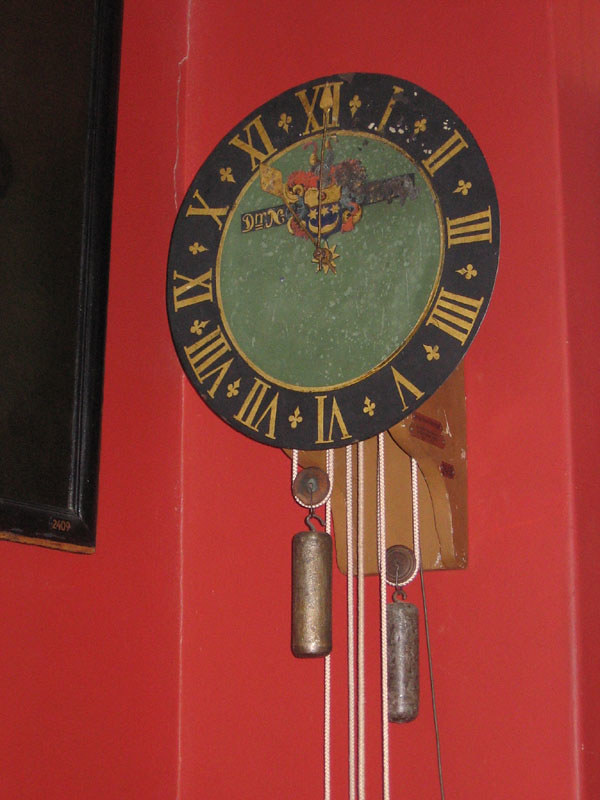An ornate, antique clock hangs on a narrow, coral-red wall, extending into a corner where it meets another section of wall painted the same color. The clock, mounted on a curved wooden base, displays a round face with an outer edge in navy and an inner section in a mottled greenish-gray, reminiscent of robin's egg blue. The clock face features Roman numerals in gold around the navy border, and two thin, brass-colored hands indicating the time as 11:01. An elaborate coat of arms design, with gold stars on a blue field, decorates the top section of the clock. Below the clock face, pendulums or cylindrical bells hang on white cords. To the left, partially visible, is a black-framed piece, possibly a mirror or a poster, with the number "2409" inscribed in gold letters at its bottom. The paint on the wall shows some cracks, adding to the vintage atmosphere of the scene.